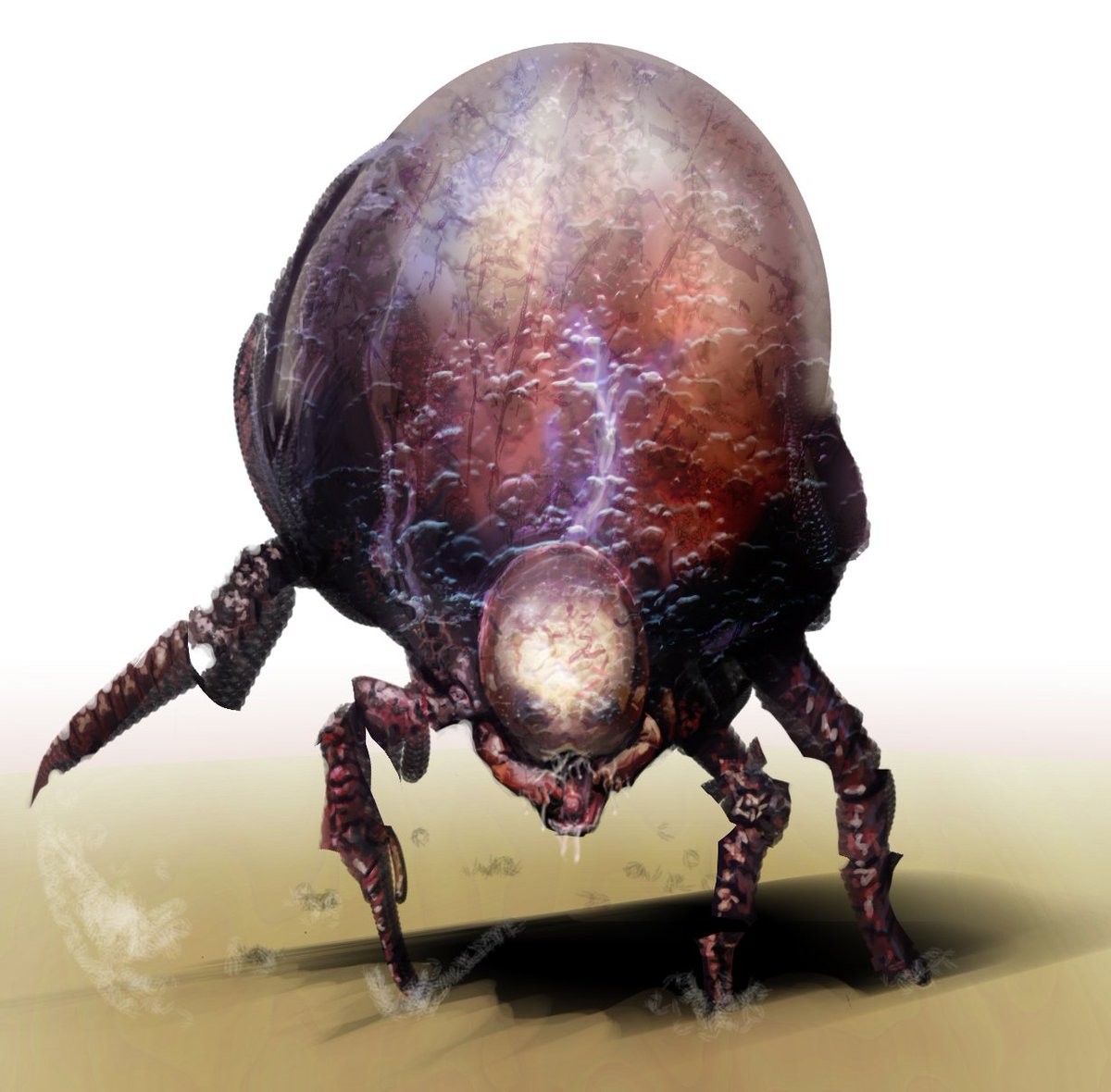The image depicts a highly detailed, four-legged creature that resembles a blend between an insect and an otherworldly monster. This creature has an enormous, egg-shaped hump on its back, which is significantly larger than its head and legs combined. The hump is marked with veins, stains, and possibly visible blood vessels, giving it a semi-transparent, organic appearance. The creature's head is smaller yet also egg-like, featuring a shiny, whitish surface with brown and reddish tones. It lacks eyes, and its gaping mouth reveals dripping saliva, with two of its front claws or hands reaching into it. The creature stands on three of its four long, spider-like legs, with the front left leg lifted as if in mid-stride. The surface it stands on is beige-yellow and appears to be dusty, casting a dark shadow beneath the creature. The background of the image is predominantly white, emphasizing the creature’s startling and grotesque details. The overall impression is that this illustration is a piece of concept art for a science fiction or horror setting, depicting an alien or monstrous insect that is both fascinating and repulsive.